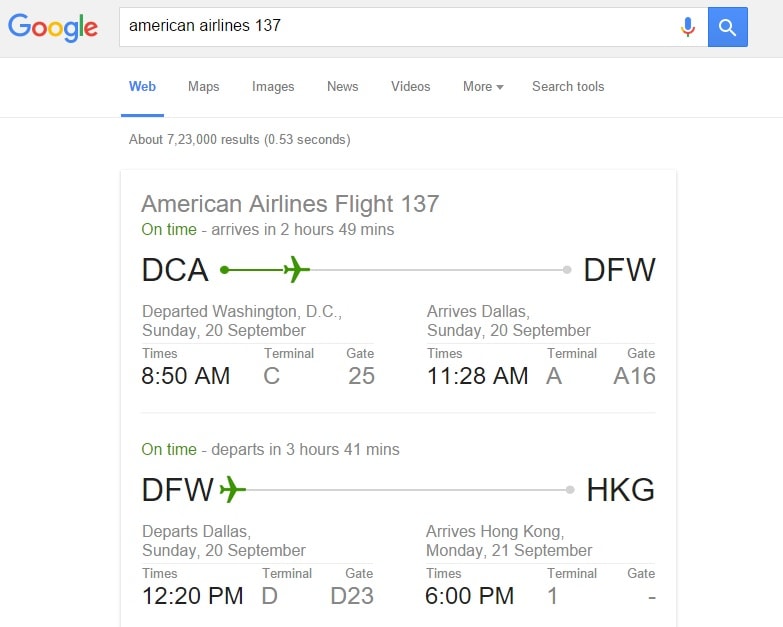The image is a vertical screenshot from a Google search results page, primarily with a white background. At the top of the image, there is a gray box featuring the Google logo in its traditional colorful design, alongside a white search bar. Inside the search bar, the text "American Airlines 137" is typed in black font. To the right of the search bar, there are two icons: a microphone and a blue magnifying glass indicating the search function.

Directly below the search bar, the options for "Web", "Maps", "Images", "News", "Videos", "More", and "Search tools" are displayed. The "Web" option is highlighted in blue and underlined, signifying that it is the currently selected category. A thin line separates these options from the search results.

Underneath this line, the page displays the total number of search results and the time taken to generate them, enclosed within parentheses. Following this, there is another thin bordered box, open at the bottom, which provides detailed flight status information. 

In the gray text, the title "American Airlines Flight 137" is displayed. Below it, in green, the status "on time" is indicated, along with an estimated arrival time of "2 hours 49 minutes."

A simple graphic shows a plane travelling from DCA (Ronald Reagan Washington National Airport) to DFW (Dallas/Fort Worth International Airport). The image includes details such as the departure date, time, terminal, and gate number, along with the expected arrival information at DFW. Additionally, the status and details for the subsequent flight from DFW to HKG (Hong Kong International Airport) are provided, including whether it is on time and the corresponding flight numbers and dates.